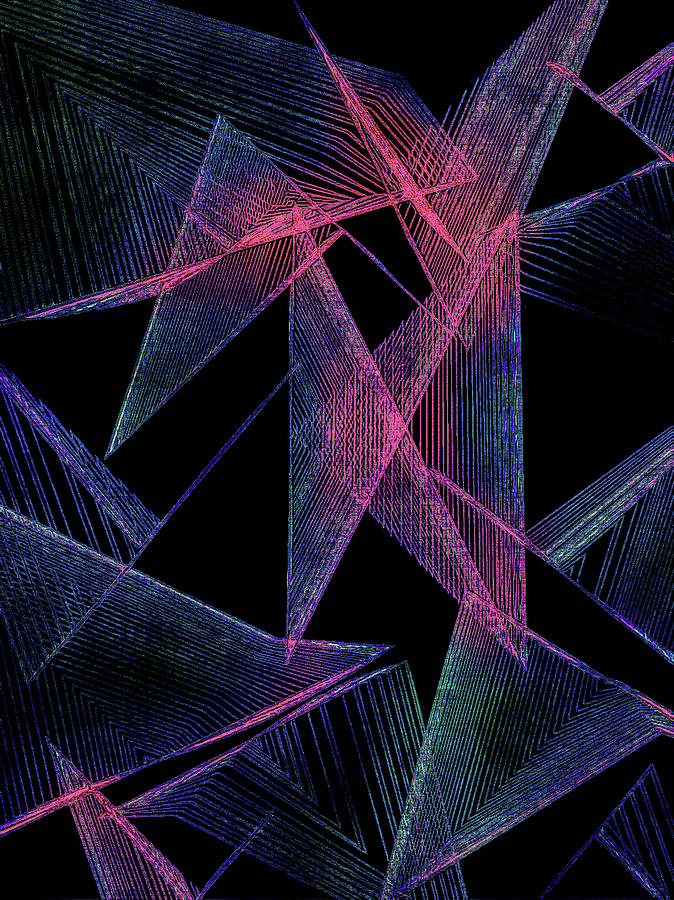This image depicts an art poster set against a black background adorned with thin, transparent lines forming intricate geometric shapes. Predominantly, these shapes are angular, consisting largely of overlapping, non-equilateral triangles, creating a complex, net-like texture. The lines, rendered in an array of colors including pink, blue, purple, green, and indigo, vary in their orientation and positioning, contributing to a dynamic, almost three-dimensional appearance. The center of the composition features more interconnected shapes, while towards the edges, the triangles are more dispersed. There is no text present on the poster, allowing the vivid interplay of colors and shapes to take center stage.